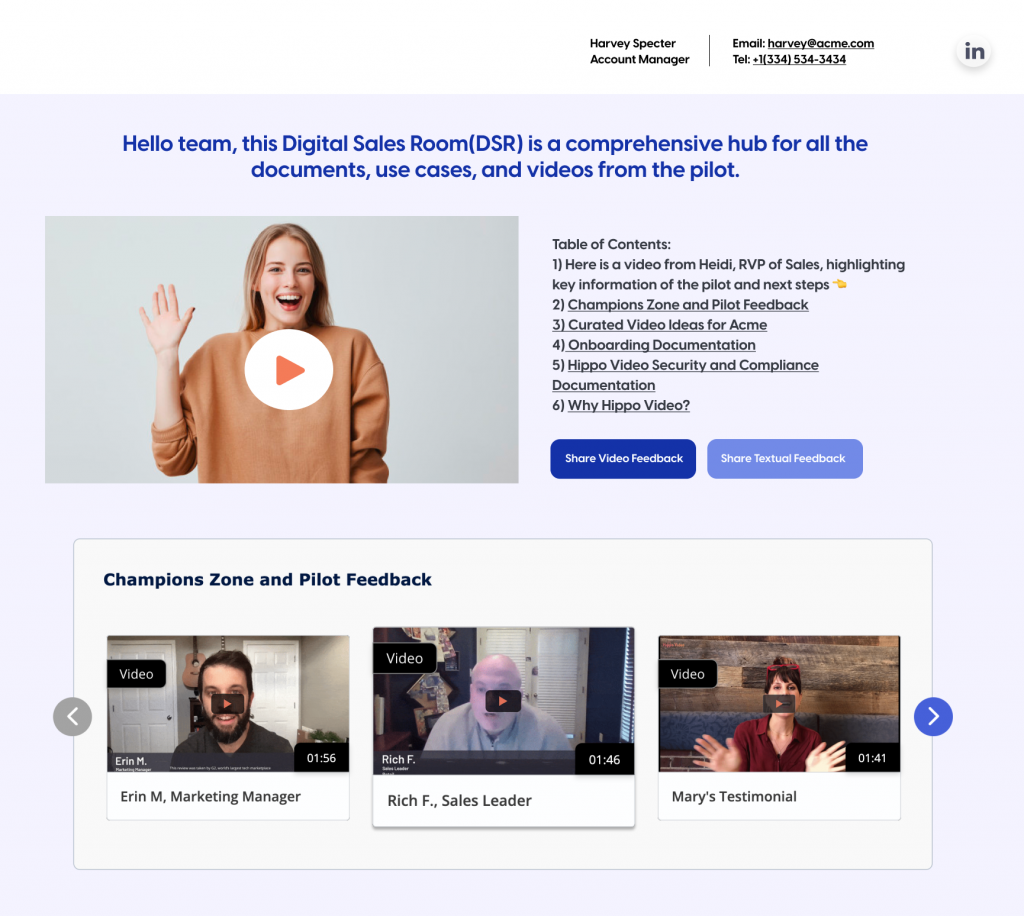The screenshot is divided into two main sections. The upper section has a white background with centrally aligned text that reads "Harvey Specter" followed by the title "Account Manager." To the right, a vertical black line separates this information from contact details. On the right side of the line, the email address is listed above the telephone number. Further to the right is the gray LinkedIn logo.

The lower section features a light blue background. At the top, in centered blue text, it reads: "Hello Team, this Digital Sales Room (DSR) is a comprehensive hub for all the documents, use cases, and videos from the pilot." A few lines down, on the left, there is a clickable square that contains a video still; it shows a woman in a sweatshirt raising her hand in greeting. To the right of the video, there is a Table of Contents listed in black text, comprising six items.

Below the Table of Contents are two buttons: the left button is dark blue with "Share Video Feedback" written in white, and the right button has a blue-gray background with "Feedback" written in white. At the bottom of the screenshot, there is a white rectangle with "Champion Zone and Pilot Feedback" written in black in the top left corner. Below this heading are three squares, each containing clickable video thumbnails.